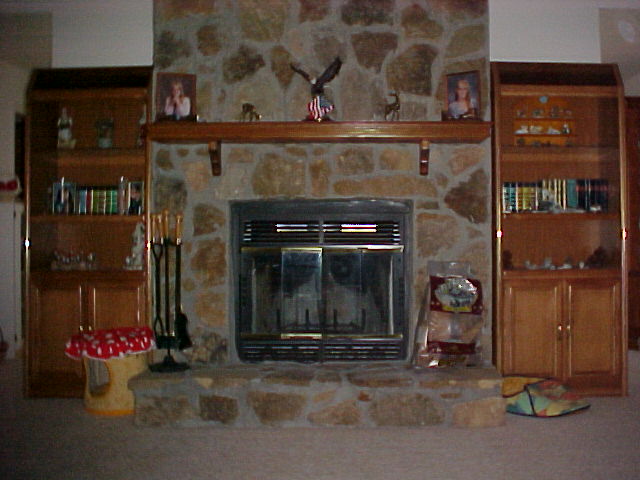The photograph captures the interior of a home, showcasing an entire wall dominated by a grand stone fireplace with a glass cover. The fireplace, made of large tan and brown irregular stones set in gray mortar, features a black border and grill. Although no logs or flames are present inside the fireplace, there is a bag of firewood to its right, suggesting it may be wood-burning. On the left, a set of wrought iron fireplace tools stands upright in a rack.

Above the fireplace, a wooden mantel displays two school day photographs of teenagers, flanked by golden animal statues, with a prominent bald eagle statue holding an American flag taking center stage. On either side of the fireplace are matching wooden shelves, filled with an eclectic mix of books, CDs, small statues, and rocks. Each shelving unit also includes small cabinet doors at the bottom, which are closed and subtly hidden from view. The room itself features a brown rug and a notable object in front of one shelf: a small piece of furniture draped with a red tablecloth, which upon closer inspection, appears to be a cat box with an opening for a feline to sleep inside. The detailed and cozy setting reflects a personalized and well-loved living space.